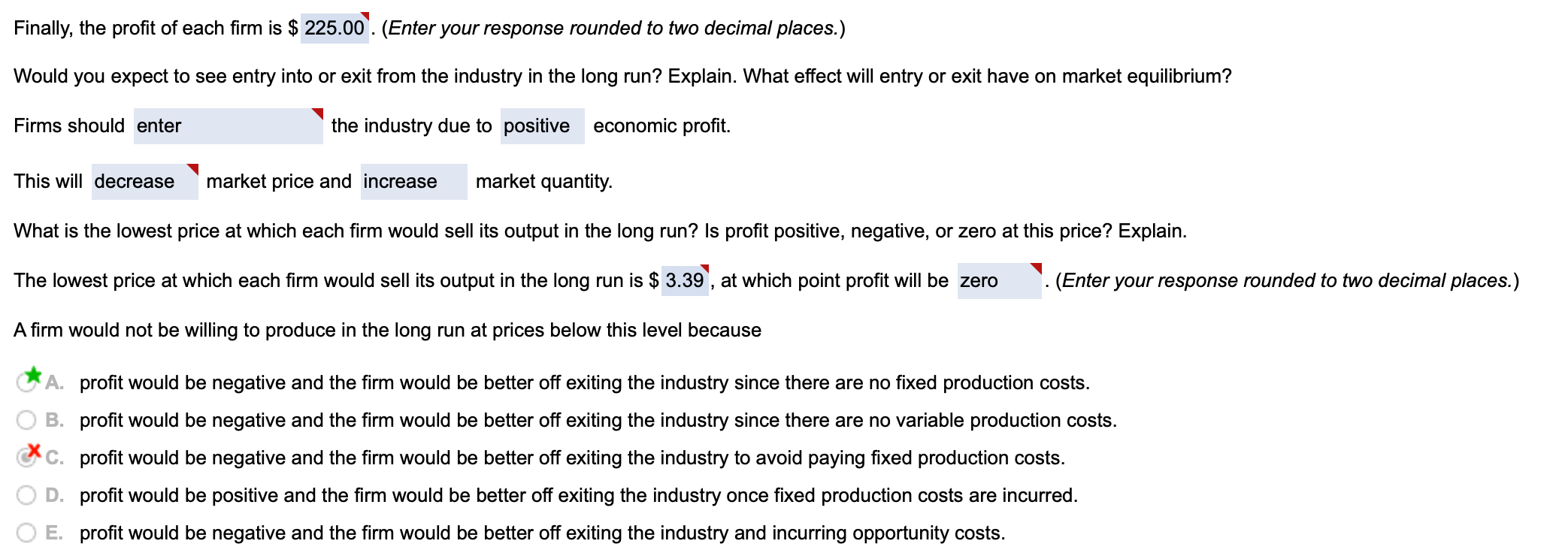The image features an excerpt from an economics or math class worksheet that provides information about firms and their profits. The background is white with black text prominently displayed, making it easy to read. The text on the worksheet includes the following content:

"Finally, the profit of each firm is $225. Enter your response rounded to two decimal places. Would you expect to see entry into or exit from the industry in the long run? Explain. What effect will entry or exit have on market equilibrium? Firms should enter the industry due to positive economic profit. This will decrease market price and increase market quantity. What is the lowest price at which each firm would sell its output in the long run? Is profit positive, negative, or zero at this price? Explain. The lowest price at which each firm would sell its output in the long run is $3.39, at which point profit will be zero. Enter your response rounded to two decimal places. A firm would not be willing to produce in the long run at prices below this level because..."

The worksheet also provides several options for students to choose from to answer the questions listed. Within the text, there are blue-highlighted input fields where students are expected to type their responses and answers to each respective question.